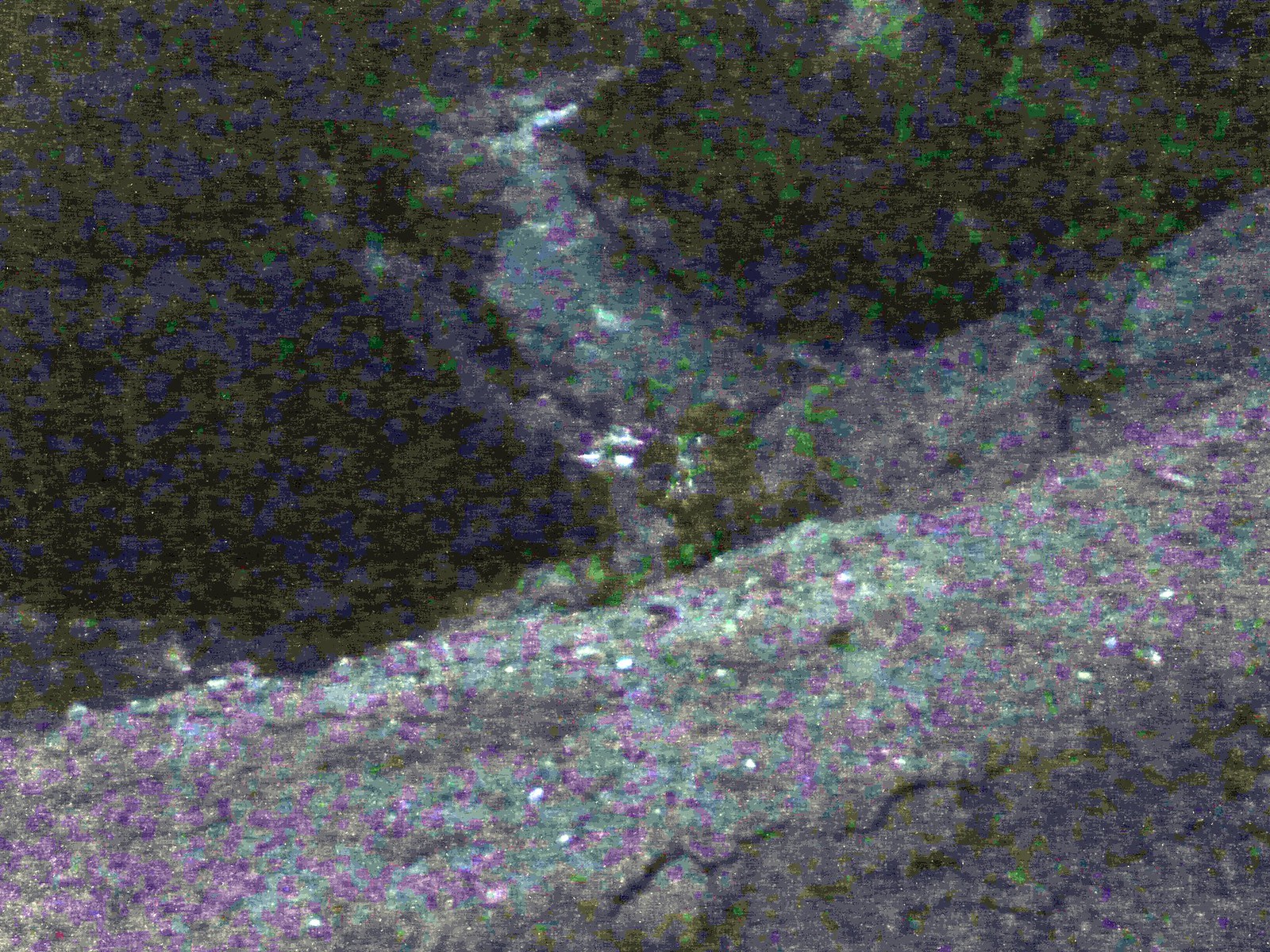This digital, pixelated and blurry image resembles a landscape scene, possibly from a computer game. Dominated by a mountainside with grayish rock dotted with pink and green specks, the image showcases diverse terrain. To the left, there's a mix of blue, brown, and green, suggesting a forested area, while the right side has more green and brown hues with touches of dark blue. Running through the center, a waterway speckled with green and purple traverses the scene. Sparse black squiggles appear in the bottom right corner. Emerging from the rock, a seemingly imaginative dragon face with purple and white horns and a brown figure underneath adds a fantastical element to the composition.